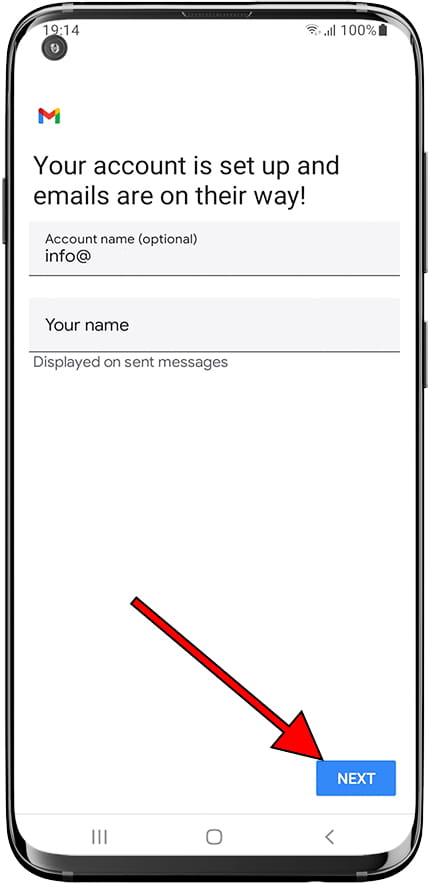The screenshot captures a mobile device's screen, showcasing the final steps of setting up a Gmail account. The device's UI reveals essential details such as the time "19:14" (military time) located at the top left, accompanied by icons displaying a strong Wi-Fi connection, data signal, and a full 100% battery charge on the top right.

The core of the screenshot shows the Gmail account setup completion page prominently featuring the colorful Gmail logo (an "M" in red, yellow, green, and blue). Below the logo, a message in black text reads: "Your account is set up and emails are on their way!" Underneath this cheerful confirmation, there is an optional "Account name" field which has been partially filled with "an info act", though the text seems incomplete.

Further down, there's another input field labeled "Your name," with a subtext that states in faded gray, "Displayed on sent messages." At the bottom of this central section, a blue "Next" button encourages the user to proceed.

Additional UI elements of the mobile device adorn the bottom of the screenshot. These include a centered navigation bar with a rounded square in the middle, three vertical lines on the left suggesting a menu button, and a left-pointing arrow on the right resembling a less-than symbol for backward navigation. A red arrow, edited onto the screenshot, points directly at the blue "Next" button, guiding the user's attention toward the final step in the setup process.